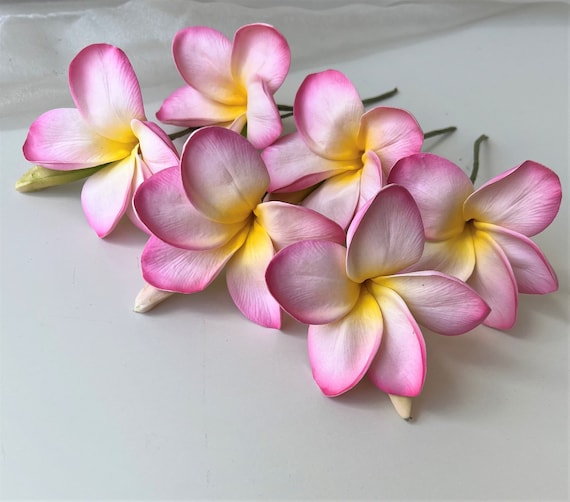This image features a bouquet of approximately six to eight flowers arranged beautifully against a plain gray background with a subtle, faint texture. The flowers, predominantly displaying shades of purple with hints of pink, have a gradient that transitions to white towards the center, culminating in a vibrant yellow at the heart. The green stems and buds are visible, some of them arching upwards towards the upper right-hand corner of the square frame. The composition exudes simplicity and elegance, emphasizing the delicate interplay of colors and natural forms against a neutral backdrop.